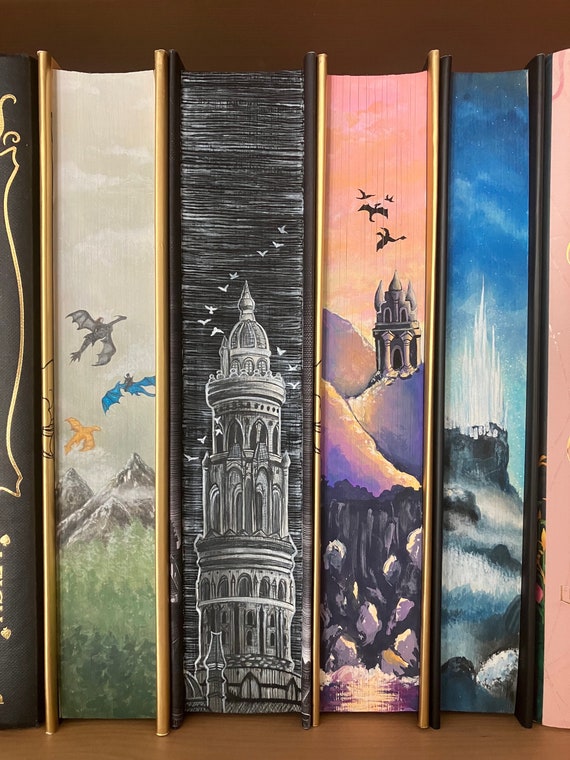The image showcases a collection of illustrated books stacked vertically on a wooden surface. The visible sides of these books, typically the pages, are intricately painted with detailed fantasy scenes. The leftmost book, partially visible, features a black cover adorned with yellow or gold designs. Next to it, a fully visible book displays a vibrant scene of three dragons — grey, blue, and yellow — soaring over green trees and mountains. Toward the middle, another book presents a majestic grey monument or tower with a dome, surrounded by white birds against a dark grey sky. Another book to the right depicts a dramatic scene of flying dragons, either black or grey, over a grey castle or fort, with striking purple mountains and rocks at the base. The rightmost book illustrates a fort-like structure perched on a cliff, with a mesmerizing blue light beam emanating from the tower into a clear blue sky. The overall setting has an educational or illustrative style, highlighting the artwork and attention to detail on the edges of the book pages, rather than the spines.